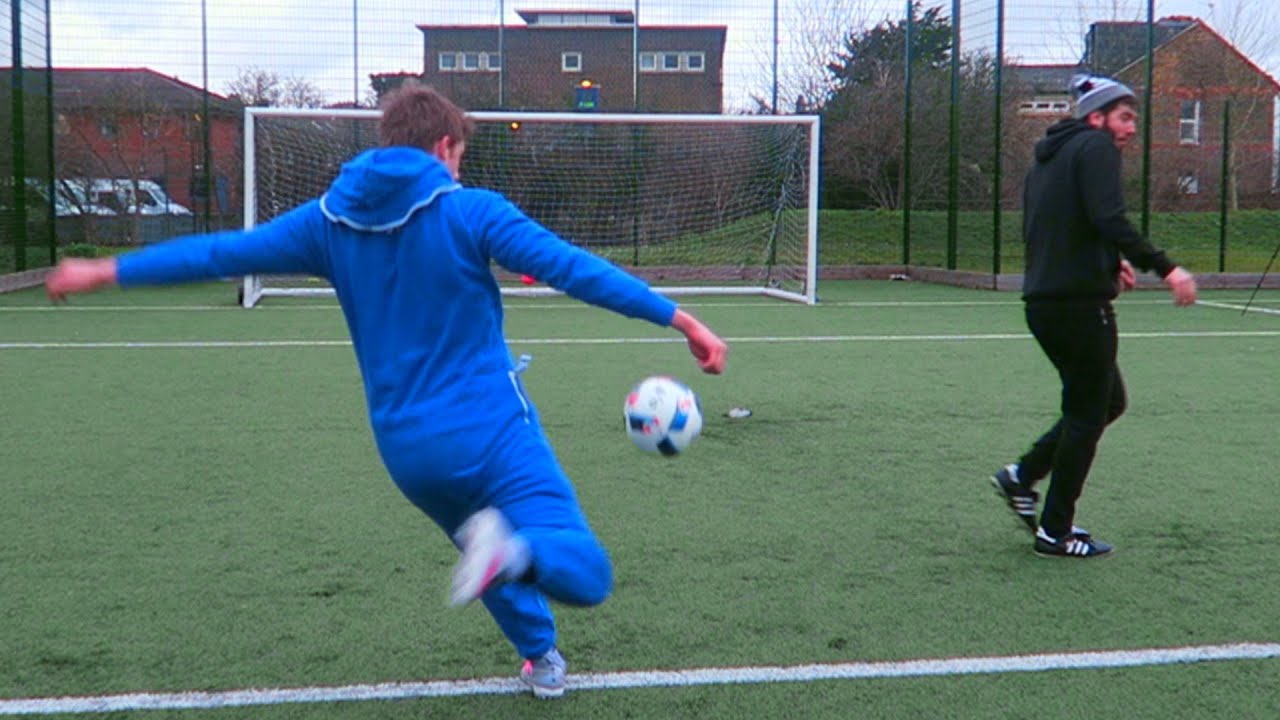The image captures an urban soccer field nestled within a residential area, surrounded by brick apartment buildings in shades of medium to dark brown and red. Each building features a mix of windows, adding to the charming residential atmosphere. The soccer field itself is enclosed by a tall wire fence, nearly the height of the buildings, effectively preventing stray soccer balls from hitting the structures.

In the center of the field, a white man clad in a blue tracksuit or sports jersey, paired with white shoes, is captured mid-action. The soccer ball is in motion, indicating that he has either just kicked it or is about to. His posture and the trajectory of the ball suggest it is headed straight towards the goal, with no immediate obstacles in its path.

Standing a bit farther away, another man, dressed in a gray hat, black sweatshirt, black track pants, and soccer shoes, is positioned with his back towards the kicker. He appears tense, crouched slightly, as if bracing himself for the incoming ball, perhaps to avoid being struck.

Overall, the scene vividly portrays a moment of intense action on the soccer field, set against the backdrop of a bustling residential neighborhood.